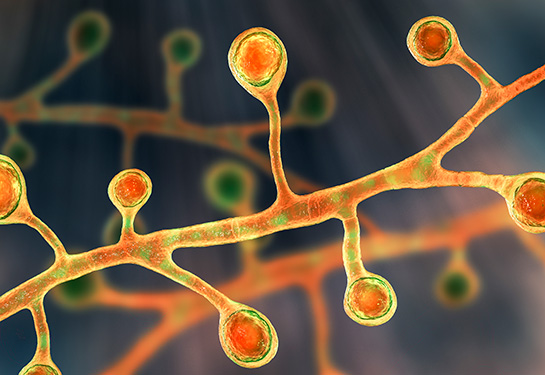The image depicts a close-up, microscope-like view of an intricate, living structure that bears a resemblance to a plant stem with cellular characteristics. The primary focus is an orangish and green stem that diagonally stretches from the bottom left to the upper right of the image. This main stem has smaller branches extending vertically up and down, each ending in round, circular nodules with green rims and orange centers. Some areas of the nodules appear to be highlighted with a faint yellow glow, suggesting an illuminated or reflective quality.

Two additional, similar structures can be seen blurred in the background, contributing to the image's depth. The backdrop itself is a mix of dark blue, black, and purple hues, with beams of light radiating from the top left, enhancing the mysterious, almost alien-like appearance of the scene. The translucent, almost ethereal colors and detailed textures suggest a blend of biological and fantastical elements, creating an intricate, otherworldly visualization.